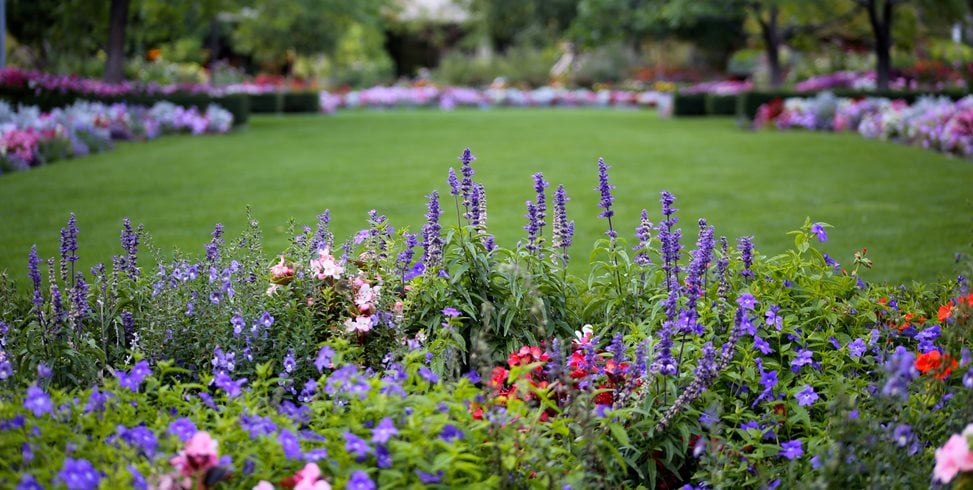This is a daytime color photograph capturing the lush environment of a public park or arboretum. In the foreground, a vibrant array of wildflowers bursts with color, including tall lavender flowers, long purple blooms, smaller round purple flowers with white centers, and vibrant red, pink, and white flowers. The flowers are nestled among green leaves, creating a rich tapestry of nature's beauty. The centerpiece of the image is an expansive, well-manicured grassy lawn without any dry patches or weeds, providing a serene green expanse. Surrounding the lawn are various gardening beds filled with a multitude of flower species in different colors—pink, white, red, and purple dominate the scenery. In the background, rows of flowers continue to adorn both sides and distant sections of the park, bordered by hedges that lead off to the left and right. Trees and the roof of a building are faintly visible in the distance, completing this picturesque outdoor scene.